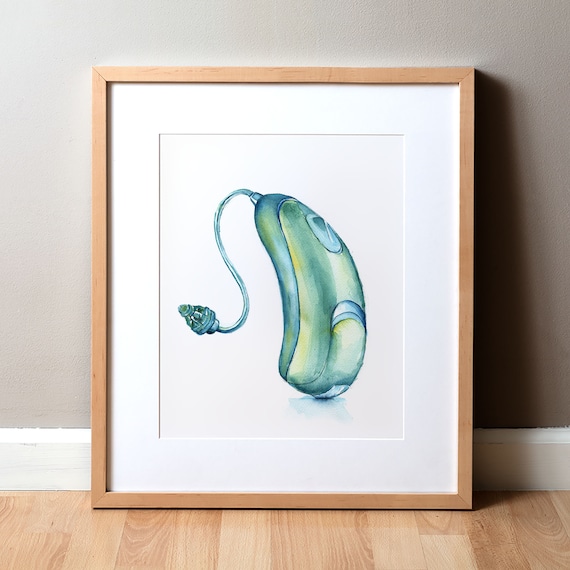The image is a vertically oriented, rectangular photograph encased in a sleek, light wooden frame that might resemble one from Ikea. The frame includes a white mat that surrounds a piece of white paper featuring an abstract drawing. Dominated by greenish-teal hues with touches of purple, blue, yellow, and white, the artwork vaguely resembles a computer mouse or an electric razor. At the top of this shape, a short wire extends, possibly ending in an ambiguous power jack or connector. The framed image is leaning against a grayish-beige wall, which casts a faint shadow on the light-colored hardwood floor beneath it, adding to the minimalist aesthetic of the scene.